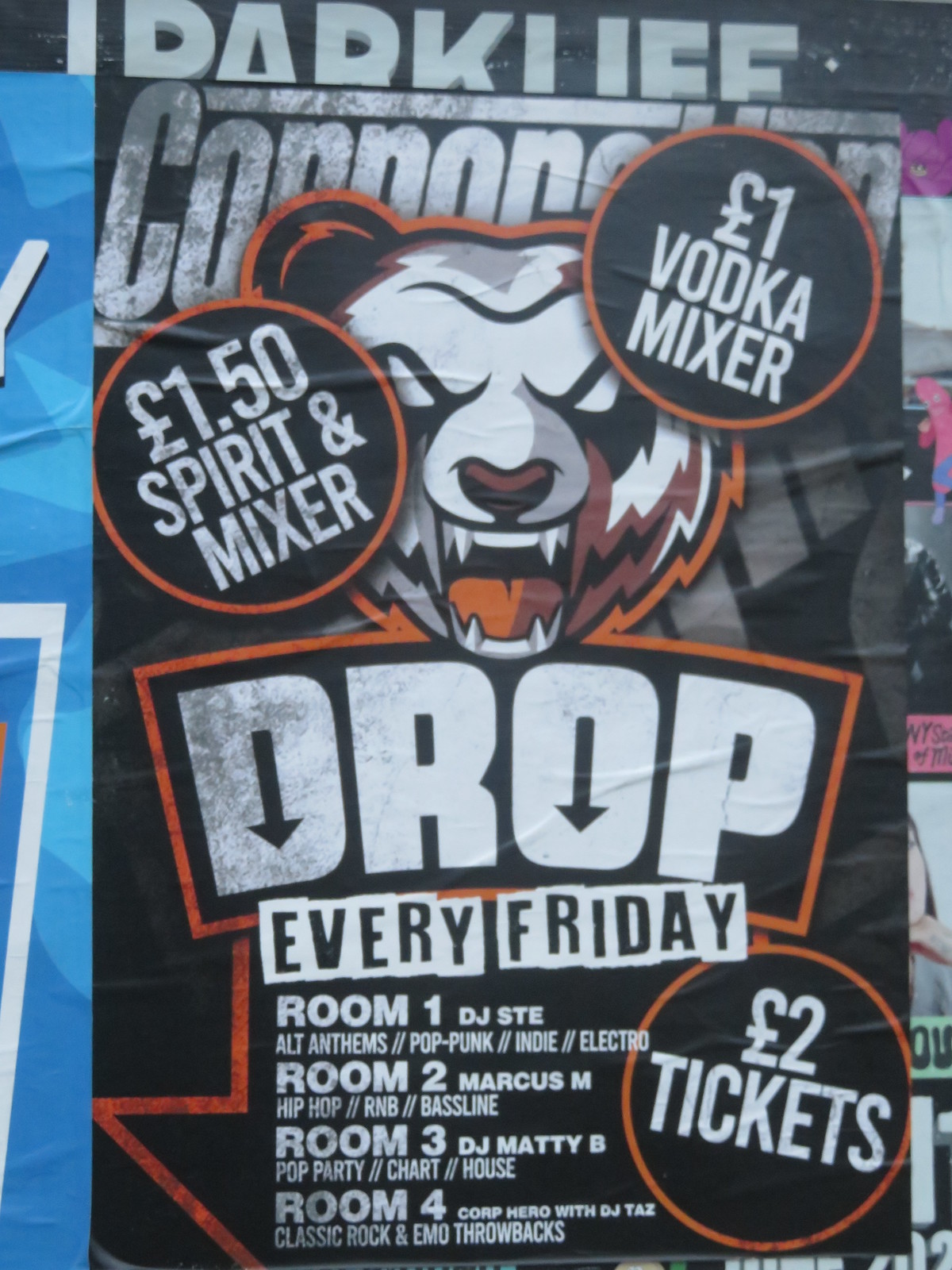This image is an advertisement poster primarily using white, orange, brown, and black colors with muted maroon highlights on a dark background with some gray elements. At the top of the poster, there is a prominently displayed snarling bear logo, which might be a panda bear with visible fangs. To the left at the top, there's a circle with a black background that states "1.50 Spirit and Mixer." Another circle on the upper right near the bear's right ear says "1 Pound Vodka Mixer." Centrally located, there is an arcing text with "DROP" in a stylized font featuring downward arrows incorporated into the "D" and "O." Below, the outlined black text says "Every Friday." 

The poster details the events across different rooms: 
- Room 1: DJ STE (alt anthems, pop punk, indie, electro)
- Room 2: Marcus M (hip-hop, R&B, bassline)
- Room 3: DJ Matty B (pop, party, chart, house)
- Room 4: Core Hero with DJ Taz (classic rock, emo throwbacks)

At the bottom right corner of the poster, it mentions "2 Pound Tickets." This poster appears to advertise a recurring Friday event, likely at a club, featuring various music genres and DJs.